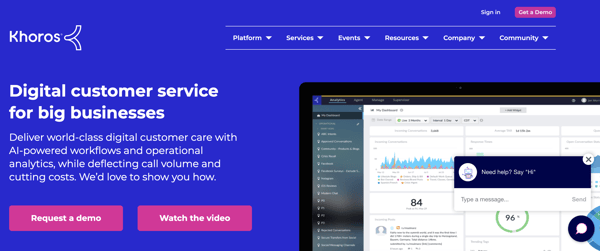The image features a predominantly blue rectangle. At the top right corner, there is a "Sign In" option, followed by a pink rectangle that reads "Get a Demo." On the left side, the logo "KHOROS" is prominently displayed in white letters. Adjacent to the logo is a white ribbon, similar in design to the breast cancer awareness ribbon. Below this, a bold white tagline states, "Digital Customer Service for Big Businesses." Underneath that, another white text explains, "Deliver world-class digital customer care with AI-powered workflows and operational analytics while deflecting call volume and cutting costs. We'd love to show you how."

Beneath this descriptive text, there are two pink buttons with bold white text: the first one says "Request a Demo," and the second one says "Watch the Video." Adjacent to these buttons, on the right side of the image, there are three layered rectangles. The largest one at the back is black, followed by a smaller white rectangle, and on top of that, a smaller black and white rectangle. 

In the topmost black and white rectangle, the white portion has a message input field labeled "Type a message," and at the top part of the black section, it displays text that appears to be "Something Help" and prompts users to "Say Hi." The rectangle also features a white circle with an "X" in its top-right corner. 

The second, middle, white rectangle features text in black, which is too small to discern, along with a small illustration resembling a graph with blue and pink lines. There's also a green circle containing the number "96" in black.

Finally, the bottom black rectangle shows a vertical list of white text along the left side, which is too small to read clearly.